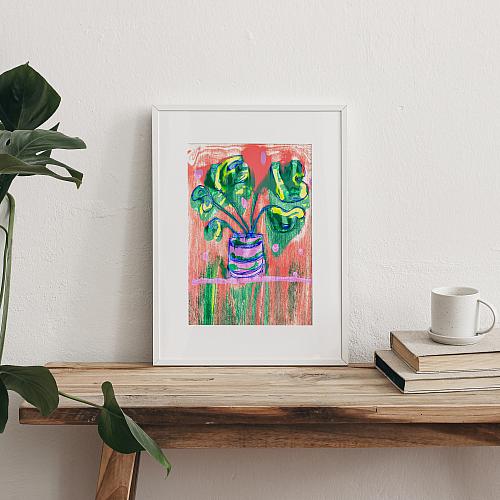A small, hand-colored painting leaning against a white wall dominates this picturesque indoor scene. The artwork sits on a wooden bench with a light wood grain finish. The painting, in a thin, possibly wooden frame with a white matte border, portrays a lilac and blue flowerpot with green leaves, accented by shades of yellow, set against a vibrant red background with green streaks. Positioned on the right side of the bench are two tan-colored books stacked on top of each other, with a white coffee mug resting on a saucer atop the books. To the left, extending towards the edge of the bench and partially obscuring the wall, is a green leafy plant, hinting at a potted flower just out of sight. The overall setting exudes a cozy and artistic atmosphere, anchored by the contrast between the bright, detailed painting and the simplicity of the wooden furniture and white walls.